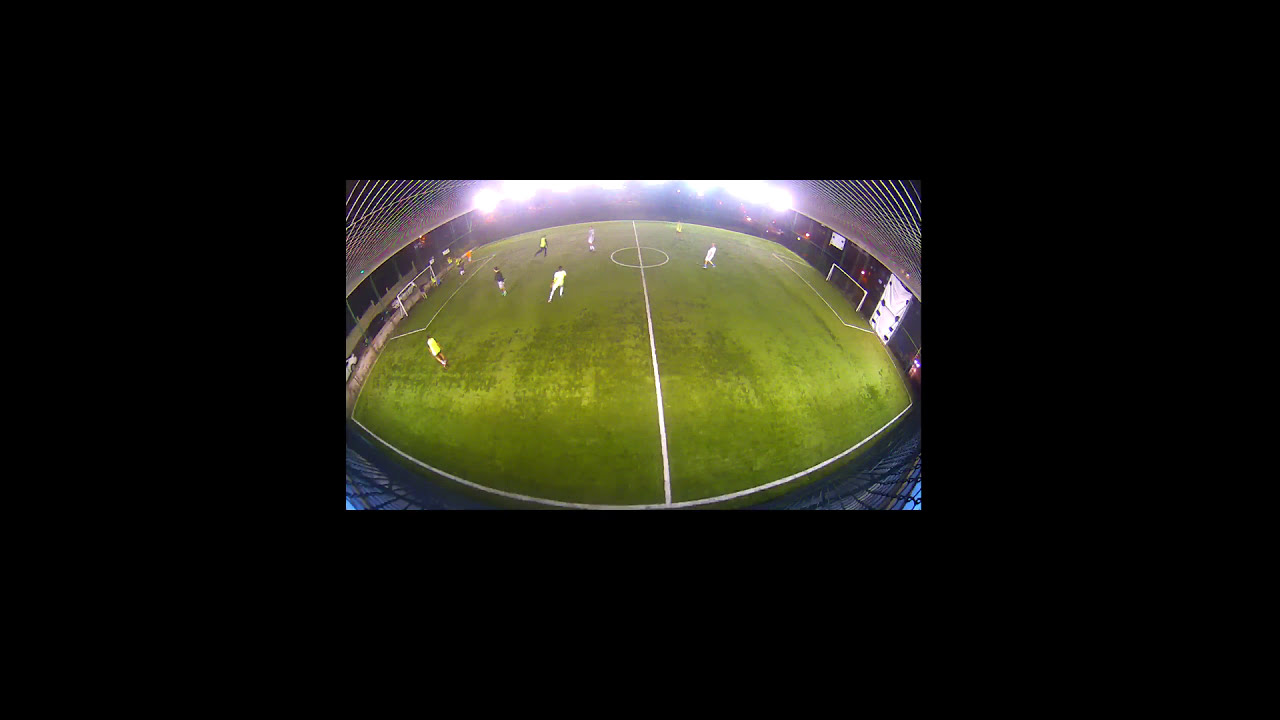The image presents an aerial view of a somewhat circular indoor soccer arena, captured with a wide-angle, possibly fisheye, lens. The green soccer field, appearing a bit worn, is illuminated by bright, centralized stadium lights against a dark backdrop suggesting it might be nighttime. The field hosts seven players: two opposing five others. The players are clad in practice attire with some in yellow, a few in white, and possibly a goalie in orange or red. The arena's structure includes black glass-like sides, and a chain-linked fence hinting at the outside. Both goals and some signs or padding are visible in the background. The ceiling edges of the arena are barely visible with some areas cut off from view, and there are no fans present, emphasizing the sense of an empty, practice-focused environment.